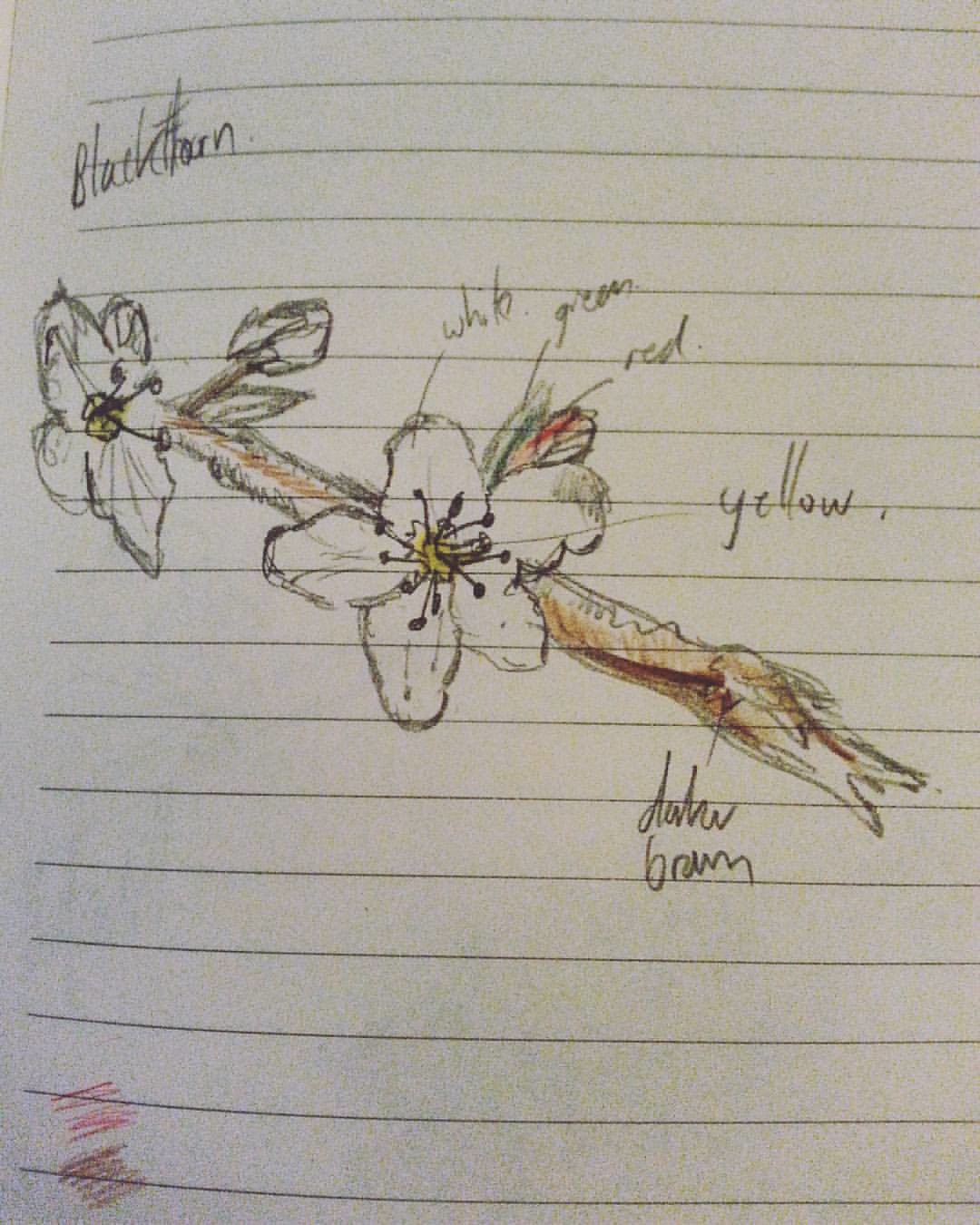In this detailed rectangular image, we observe a notebook-style piece of paper with horizontal lines, viewed from above. Sketched using colored pencils, a branch adorned with flowers extends diagonally from the upper left to the lower right. The brown branch features two white flowers outlined in black, each with a yellow center. Handwritten annotations surround the illustration: "darker brown" points to the stem or branch, while "yellow" indicates the flowers' centers. Additionally, "red, green, and white" is noted nearby. In the top left corner, the phrase "black farm" is written in pencil.